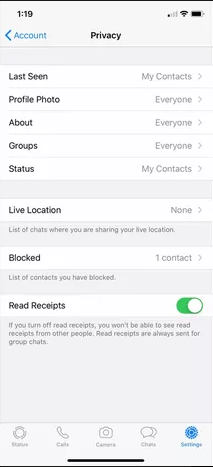**Descriptive Caption:**

The image depicts the Privacy Settings screen of an unidentified mobile application. The phone's status bar at the top shows the time as 1:19, one reception bar, a full Wi-Fi signal, and an almost full battery icon. A blue back arrow and a blue account icon are at the top of the screen. 

In the center, the word "Privacy" is prominently displayed, followed by a light gray section with options related to privacy settings. The options include:
- **Last Seen**: My contacts
- **Profile Photo**: Everyone
- **About**: Everyone
- **Groups**: Everyone
- **Status**: My contacts
- **Live Location**: None
- **Blocked Contacts**: 1

Further details explain that read receipts are currently enabled. It also notes that if read receipts are turned on, you won't be able to see read receipts from others, with the exception of group chats where read receipts are always sent.

At the bottom menu, labeled icons indicate options for Status, Calls, Camera, Chats, and Settings. The Settings icon is depicted as a blue gear, while the others are simple light gray icons.

The image appears blurry, making the text and some details hard to discern. It's not clear whether the device used is an iPhone or an Android, as the image provides insufficient clarity to confirm.